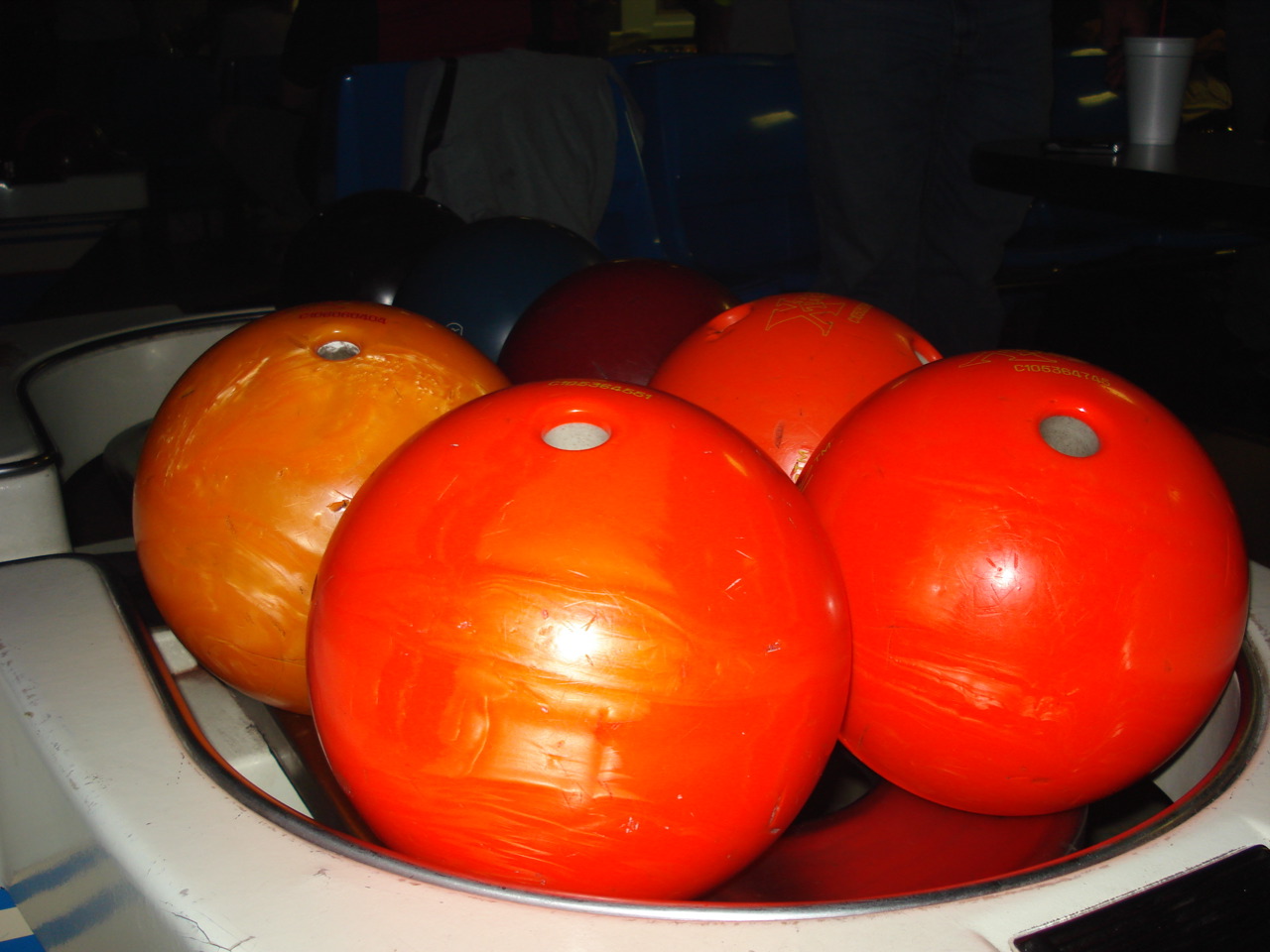This color photograph, taken with a bright flash, captures a close-up of the ball return mechanism at a vintage bowling alley. The image showcases six bowling balls nested in a horseshoe-shaped basin, which is scuffed and shows signs of an older design. In the foreground, three bright red bowling balls and one marbled orange ball are prominently visible, with their finger holes and worn surfaces catching the light. Toward the back, additional balls in dark red, blue, and black are partially obscured by shadows. The background, though dark, hints at the presence of a bowling lane environment, with glimpses of a table's edge, a styrofoam cup, and the hem of a jacket's sleeve. The overall scene has a mystical and intriguing aura, heightened by the flash's brightness and the vivid colors of the bowling balls.